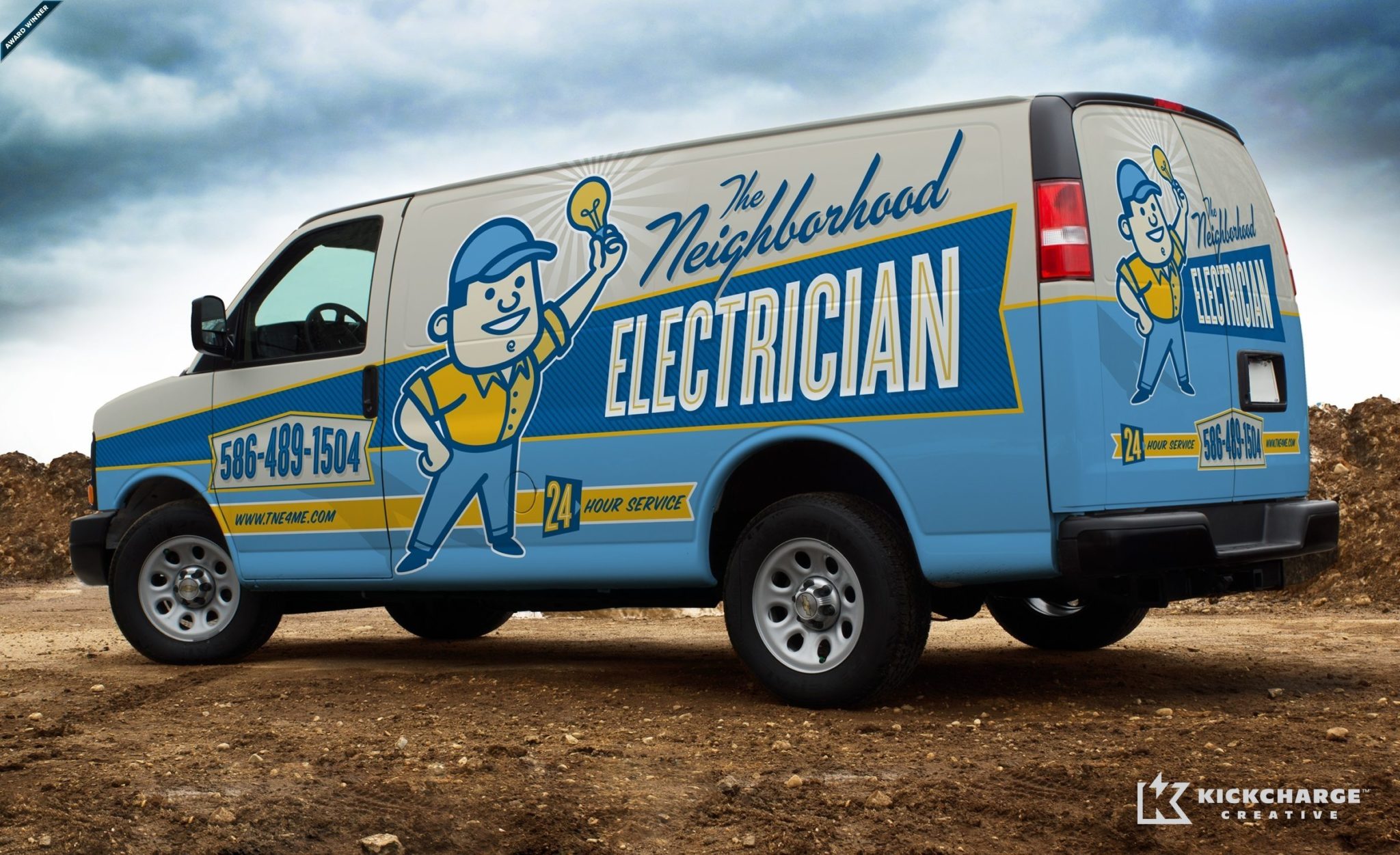In this image taken outside, a business van is prominently featured against a background of black and gray clouds set against a white sky. The barren ground is dark brown dirt intermixed with rocks. The van, primarily white with medium and light blue stripes, as well as yellow accents, showcases a detailed, colorful advertisement. The van is associated with "The Neighborhood Electrician."

On the side of the van, there is an illustration of a man in a blue baseball cap, yellow shirt, and blue pants, holding a yellow light bulb. The man's face is white with blue eyes and a blue nose, depicted in a smiling, cartoonish manner. The text "The Neighborhood" appears in blue within the white upper part of the van, while "electrician" is written in white within the darker blue area. 

Additional details include the phone number, 586-489-1504, displayed in blue on the front door. A yellow strip along the blue part of the van houses the website, www.tne4me.com, and another section reads "24-hour service" in yellow against a blue background. The back of the van mirrors these details, featuring the same cartoon man, the company name, the service hours, and the contact number. 

A logo in the bottom right corner of the van reads, "Kick Charge Creative," and a small banner at the top left corner indicates the van is an "Award Winner." The setting emphasizes the van's bright colors against the somber, cloudy sky and barren landscape.